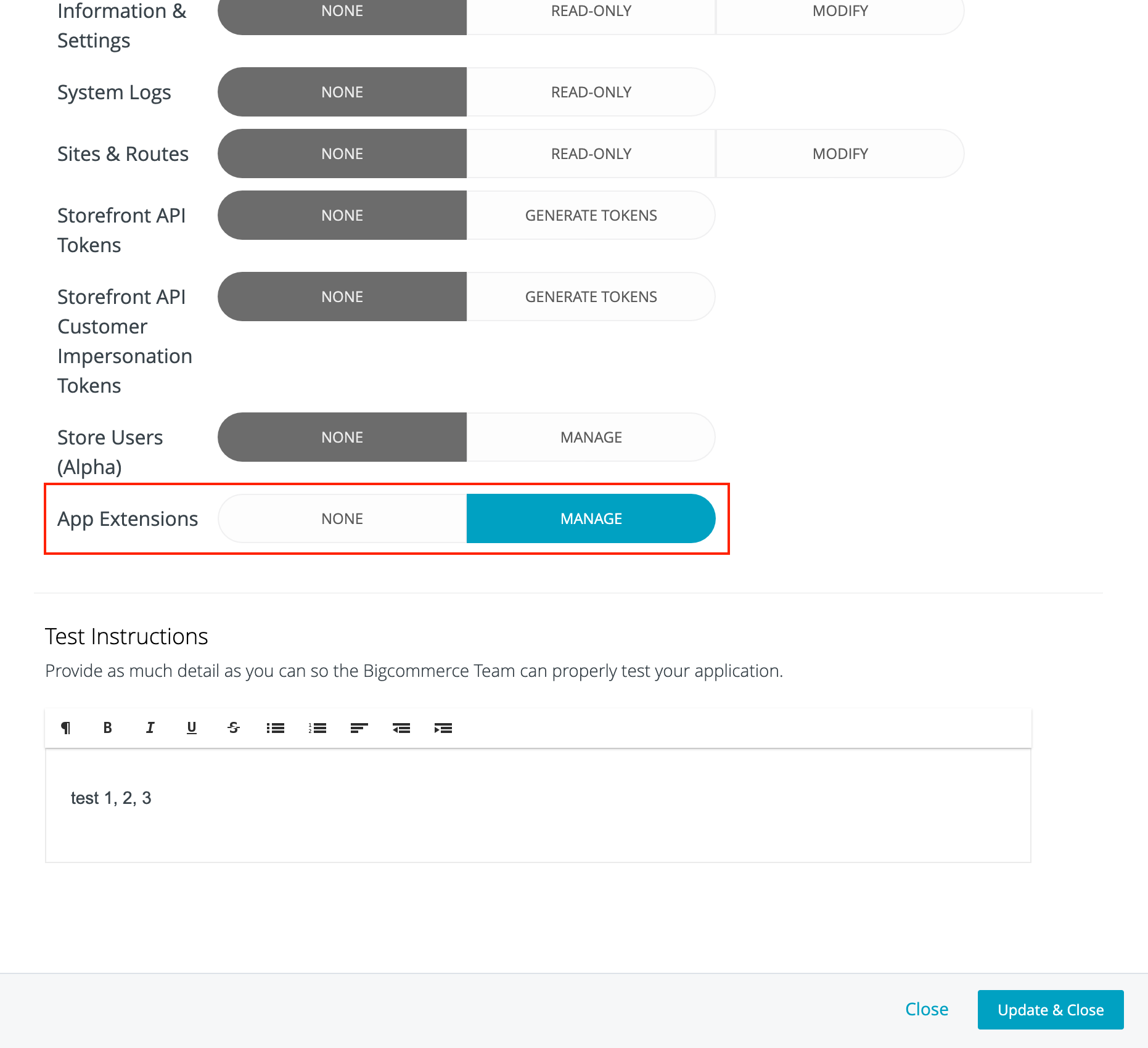The image depicts a detailed user interface screen capturing elements related to managing settings and permissions for a software application, likely related to a BigCommerce account. The leftmost column outlines different sections titled "Information and Settings," "System Logs," "Sites and Routes," "Storefront API Tokens," "Storefront API Customer Impersonation Tokens," and "Store Users." Each of these sections has an accompanying button labeled "None."

Below these sections, there is a horizontally aligned rectangle with a red border, adjacent to texts indicating "App Extensions," "None," and a blue button labeled "Manage." Further to the right, a series of labels including "Read Only," "Modify," "Read Only," "Modify," "Generate Tokens," "Generate Tokens," and "Manage" are positioned.

At the bottom of the page, a prompt reads: "Text Instructions. Provide as much detail as you can so the BigCommerce team can properly test your application." Following this guidance, several small, familiar text formatting icons span horizontally from the left edge to the mid-page. These icons include a "B" for bold, an "I" for italic, a "U" with an underline, and an "S" with a strikethrough line, among others.

Beneath these icons sits a large rectangular text box with a white background. Inside, the text reads: "Test 1, 2, 3." The entire interface shares a cohesive white background.

Finally, the bottom right corner of the page features two buttons: one marked "Close" and another labeled "Update and Close."